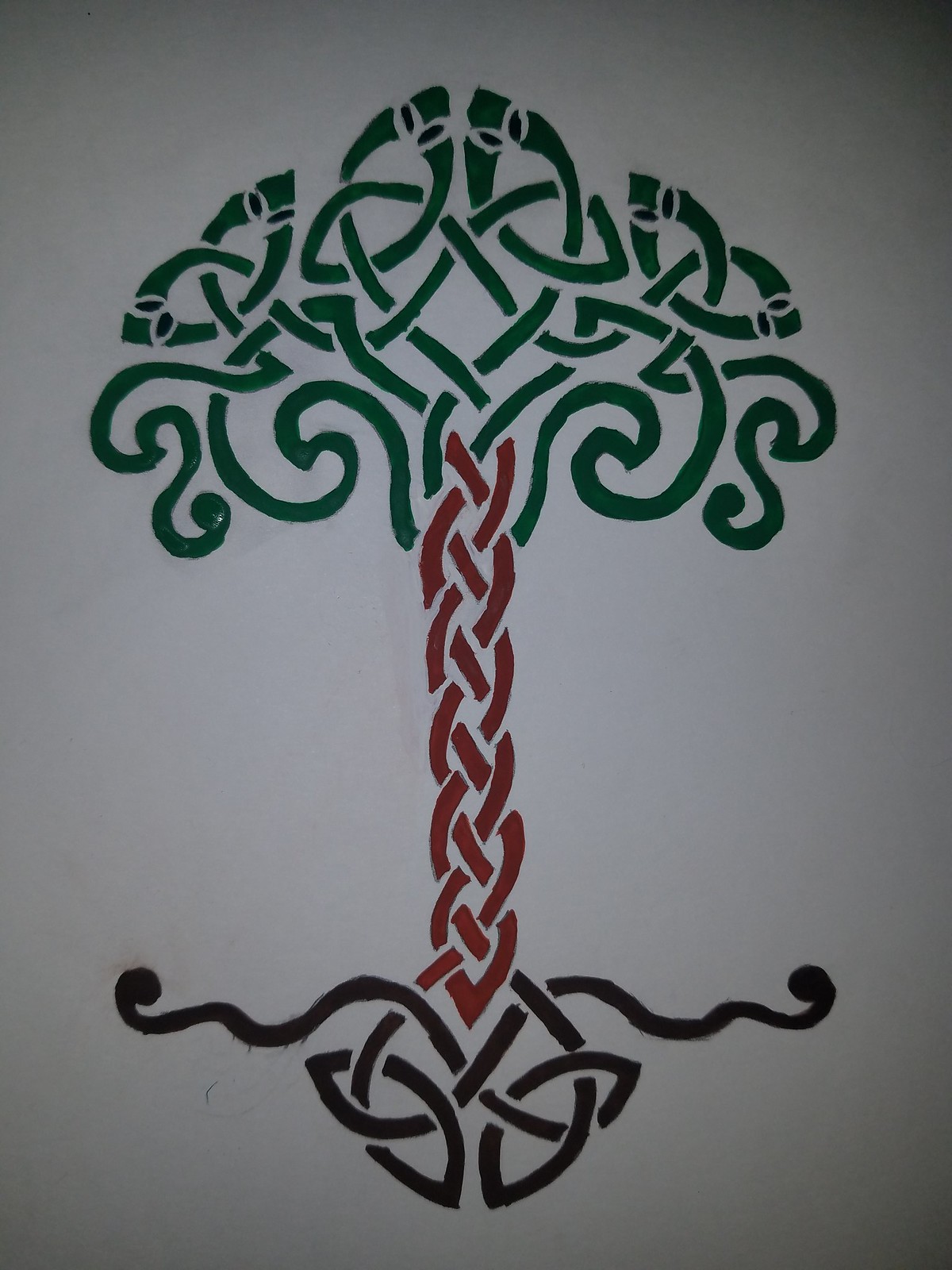The image is a detailed colored drawing of a stylized Celtic knot tree, meticulously crafted in ink on white paper. The tree's canopy is formed by intricate green Celtic knots that resemble leaves and branches, creating an umbrella-like shape. The sturdy trunk is rendered in a densely woven, reddish-brown Celtic knot that stands out vertically and transitions smoothly into the roots. These roots expand into a triangular base and are composed of darker brown or possibly black knots. Throughout the design, each section of the tree – from the leaves to the trunk to the roots – is characterized by the classic Celtic knot style, where curves and shapes interlace without touching, leaving white spaces that delineate the individual strands. This elaborate interweaving of knots imbues the tree with a sense of unity and complexity, encapsulating the timeless elegance of Celtic art.